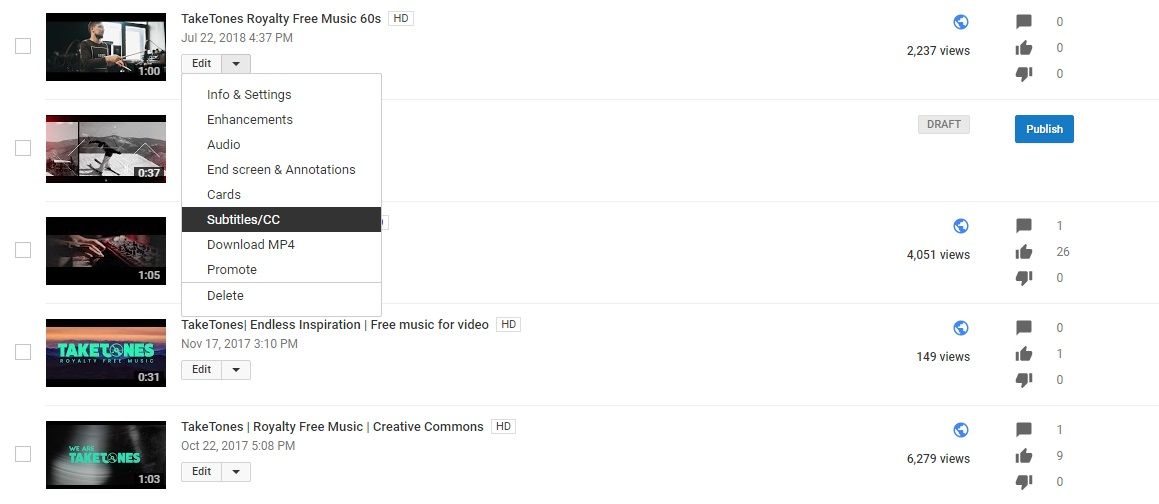In the image set against a white background, we see a detailed screenshot of a website interface. Starting from the upper left corner, there is a thumbnail image of a video featuring a young man sitting at a desk. To the right of this thumbnail, in bold gray text, is the title "Take Tones Royalty-Free Music: 60s HD." Directly below this title, in light gray text, is the date and time "July 22nd, 2018, 4:37 PM."

Adjacent to this information is a box with a pull-down menu labeled "Edit." When expanded, the menu reveals several options, all listed in gray text: "Info and Settings," "Enhancements," "Audio," "End Screen and Annotations," "Cards," and "Subtitles/CC." The "Subtitles/CC" option is highlighted in black, indicating it is currently selected. Below the highlighted option are additional buttons labeled "Download MP4," "Promote," and "Delete."

Further down, still on the left side, below the initial video option, there are thumbnails for three more videos. The second video thumbnail indicates a duration of ".37 seconds." The third video shows a length of "1 minute and 5 seconds." The fourth video down is titled "Take Tones, Endless Inspiration, Free Music for Video."

The overall design and layout are clean and organized, providing a clear and concise view of the available options and videos. The interface elements are straightforward, making it easy to navigate through different editing and management features.